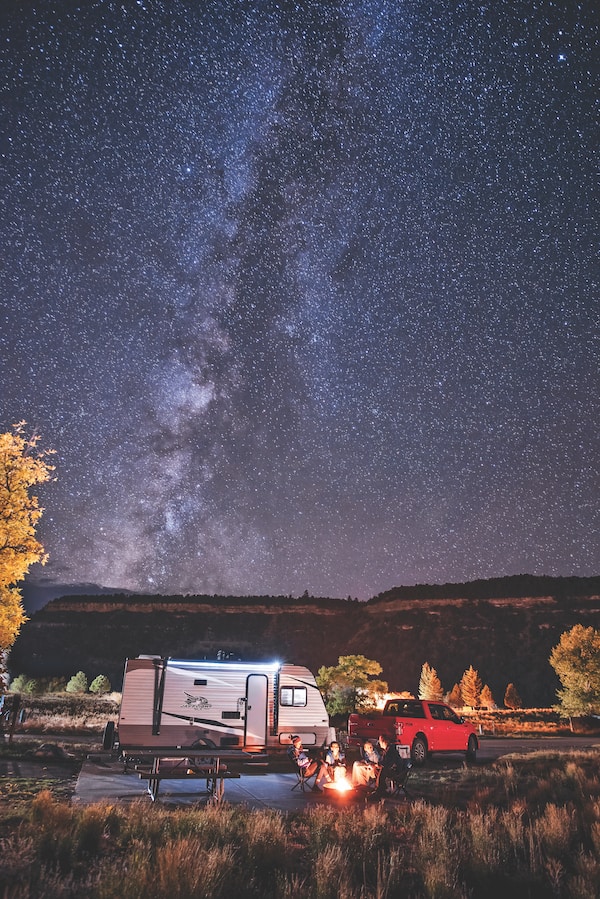In this nighttime camping scene, a group of four people is gathered around a cozy campfire, surrounded by folding chairs and a picnic table, creating a sophisticated campsite setup. They are situated near a white trailer hitched to a red pickup truck. The left side of the image features a tree with brown leaves, while the far distance reveals grassy hills and scattered shrubs, lending a slightly desert-like feel to the landscape. The sky above dominates the image with a breathtaking display of thousands of stars, creating a celestial tapestry of white and blue dots that illuminate the night with their brilliance. The scene captures the tranquil atmosphere of a night spent outdoors, enjoying the serenity and wonder of the star-filled sky.